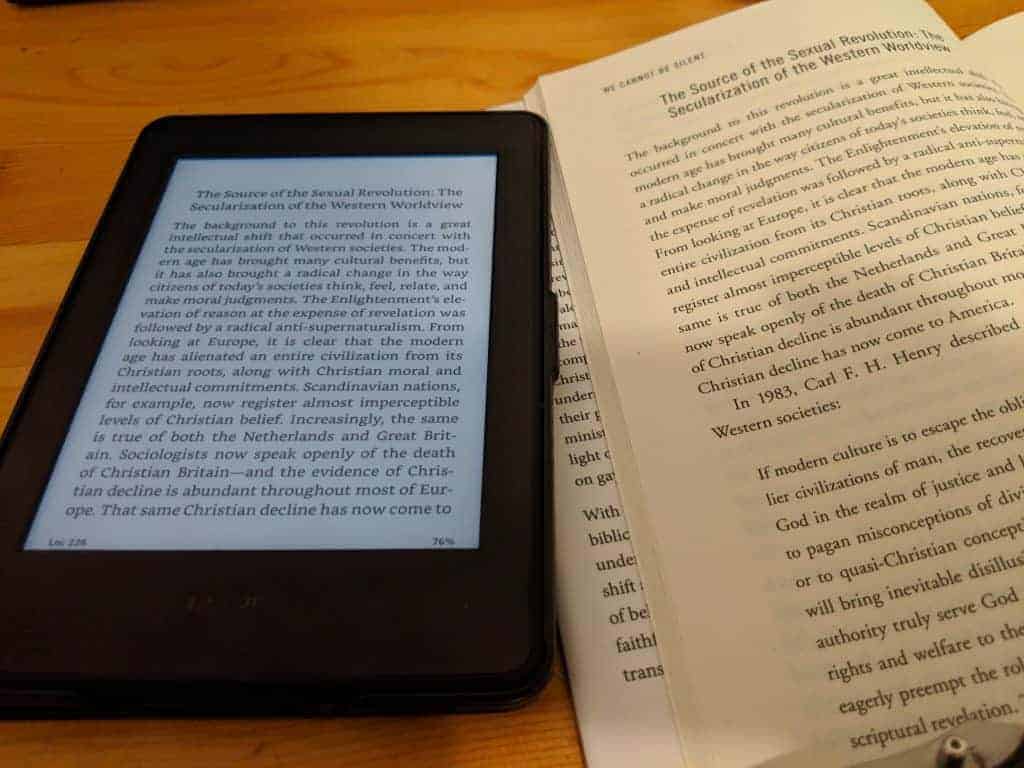The image showcases an e-book reader and an open physical book resting side by side on a light brown wooden tabletop, with visible wood grains. The e-reader, positioned on the left side of the photo, features a black frame with a white background screen displaying black text. It's reminiscent of devices like a Kindle or Nook. To its right, an open physical book reveals a page with the title: "The Source of the Sexual Revolution, the Secularization of the Western Worldview" at the top. Both the e-book reader and the physical book are aligned, sharing the same page content. The rectangular photograph is taken horizontally, capturing both devices clearly against the textured wooden surface.